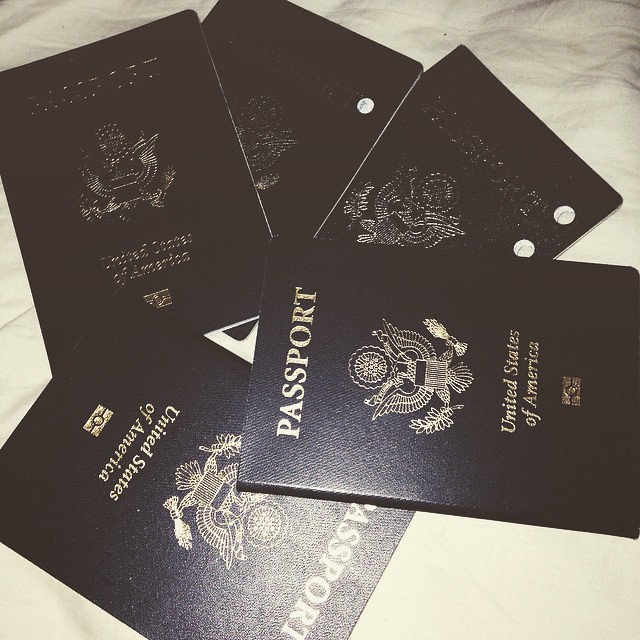This is a highly desaturated photograph depicting five United States passports arranged haphazardly, forming a loose circle. Initially blue, the lack of saturation renders the passports a pale brown hue. They rest on a pale yellow background, likely a white cloth or sheet that has been discolored by the desaturation. Among the five passports, two are punctured with holes, indicating they have been invalidated. The passports are situated without any particular order; one is positioned sideways and prominently displays "Passport United States of America." Although closely positioned, each passport can be distinguished, with one partially obscured beneath the others. This close-up photo emphasizes the texture and arrangement but does not reveal any internal details such as photographs or personal information.